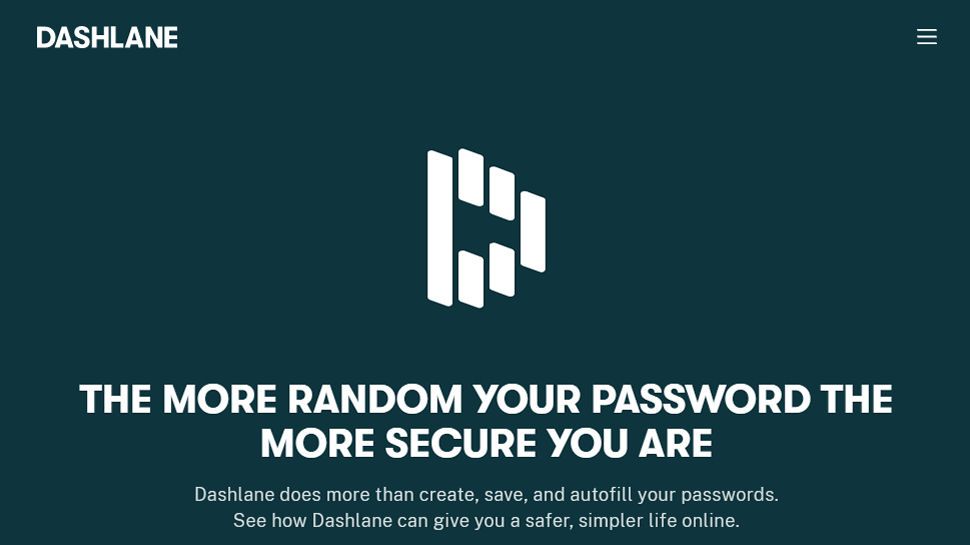A large, dark green box occupies the image, featuring the text "Dashlane" in the upper left-hand corner in white lettering. The center of the image showcases a design element with small white flashes forming the shape of a "D." Prominently displayed in bold, white typeface is the message: "The more random your password, the more secure you are." Directly below, a smaller, but still easily readable, text elaborates: "Dashlane does more than create, save, and autofill your passwords. See how Dashlane can give you a safer, simpler life online."